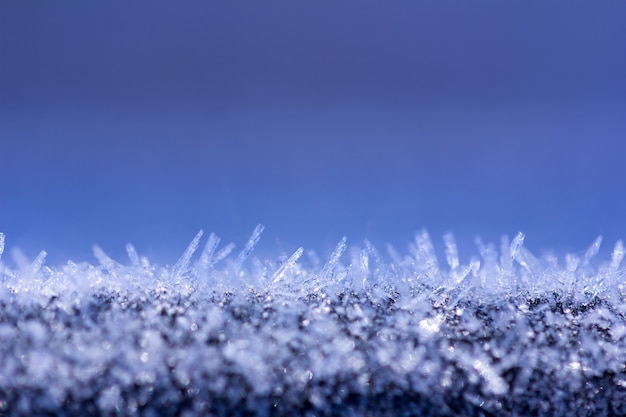This highly detailed and close-up photograph captures the mesmerizing beauty of ice crystals forming on a surface. The lower portion, making up about a quarter of the image, shows a textured, possibly metallic, surface densely adorned with tiny, fragmented ice crystals. These crystals are icy blue in color and appear to jut out in various directions, from left to right. The background transitions smoothly from dark blue at the top to a lighter blue at the bottom, providing a striking contrast that enhances the frosty details in the foreground. The perspective is extremely close, emphasizing the intricate structure of the ice. There is no text present, allowing the visual elements to fully immerse the viewer. The setting of this photo is within a rectangle format.